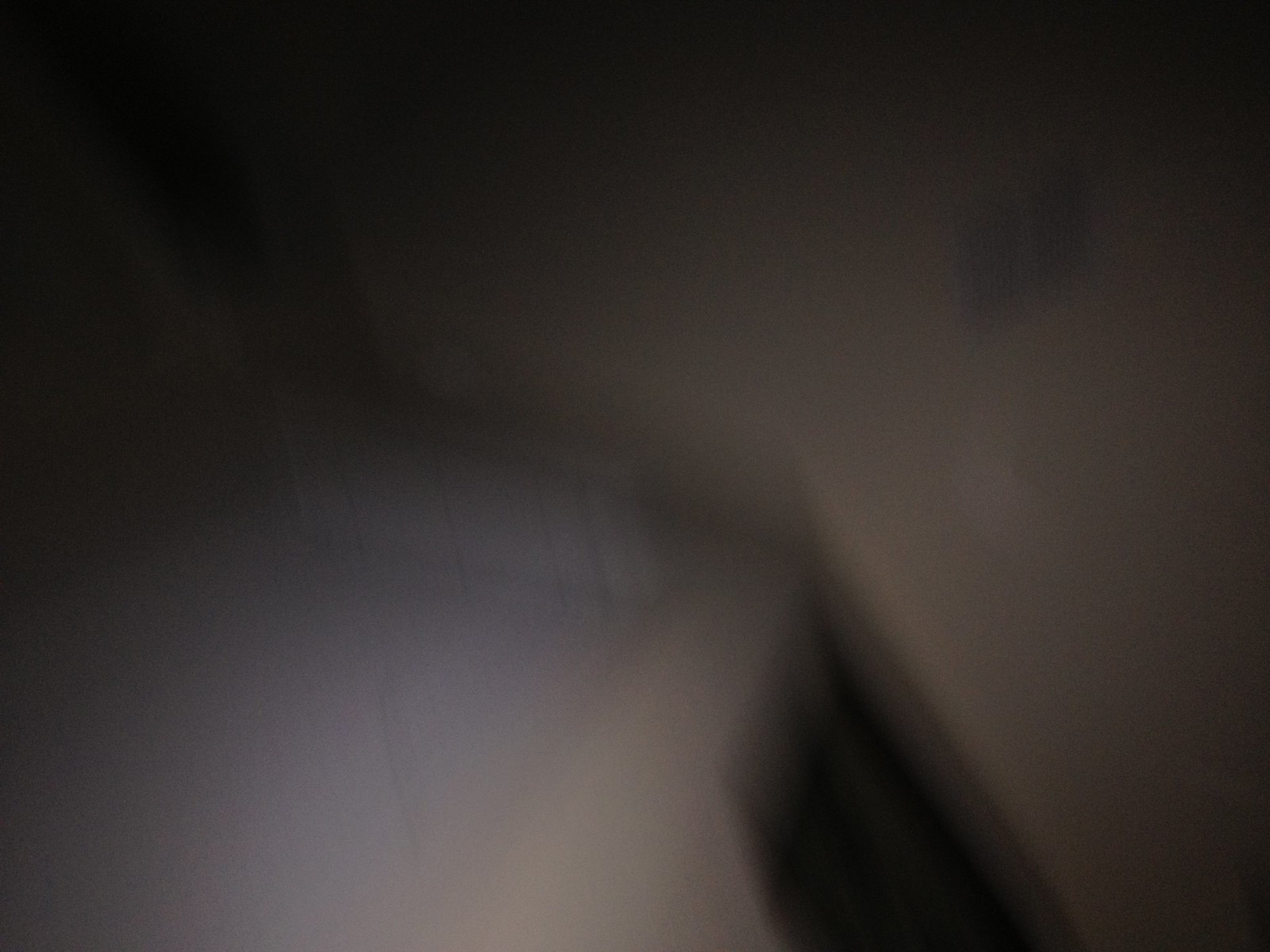This photograph presents a highly abstract and blurred composition, dominated by a gradient from black in the top left to a lighter gray in the center. The overall scene is devoid of identifiable objects due to extreme out-of-focus blurring, creating an enigmatic and ambiguous visual experience. The center is dimly illuminated, suggesting a faint source of light. In the bottom right middle, a distinct yet indecipherable black rectangular shape extends partially out of the frame, adding a touch of geometric intrigue. Additionally, a faint small square shape is barely visible in the top right corner, offering a subtle hint of structure amidst the pervasive blur. The image's overall effect is a study in abstraction and tonal contrast, leaving much to the viewer's imagination.